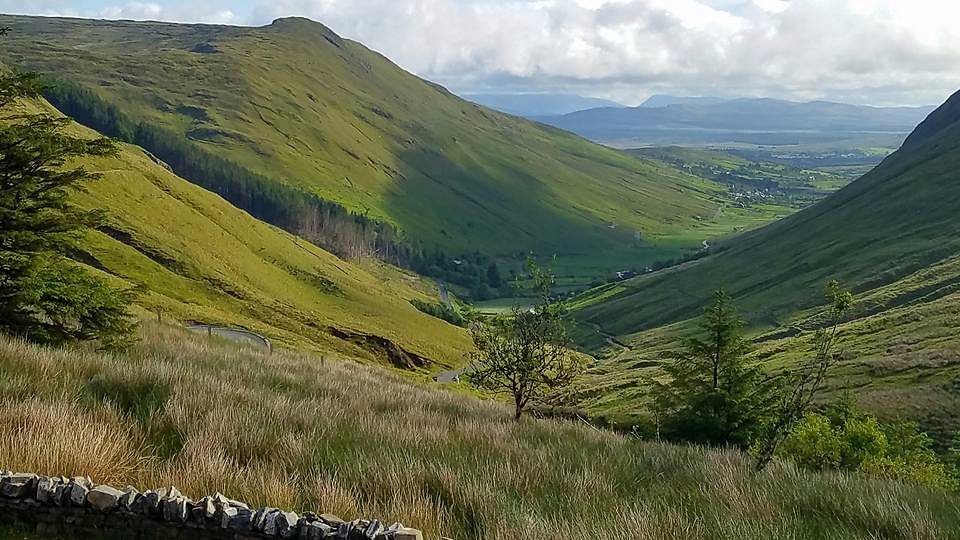This image depicts a stunning, vibrant green valley framed by gently sloping hills and towering mountains. In the foreground, on the bottom left, a short stone wall anchors the scene, partially enveloped by tall, green hay-like grasses and patches of straw-colored grass. A mixture of evergreen and deciduous trees punctuates the landscape, with pine trees spread sporadically from left to right and a stand of trees extending up a gully on the left side.

The valley itself undulates gracefully, swooping up on the sides before descending again into a cultivated expanse of green fields, likely used for hay or pasture. A wooden fence line with visible posts runs through part of the scenery. As the land flattens out in the far distance, a settlement or village can be discerned, nestled against the base of the farther, grayish mountains. Beyond the mountains, a river meanders, adding to the tranquility of the scene.

Above, the sky is filled with fluffy white cumulus clouds, allowing hints of blue to peek through, casting varying shades of shadow and light across the landscape below. The interplay of greens and shadows on the hills gives an almost mountainous appearance, contributing to the overall beauty and serenity of the view.